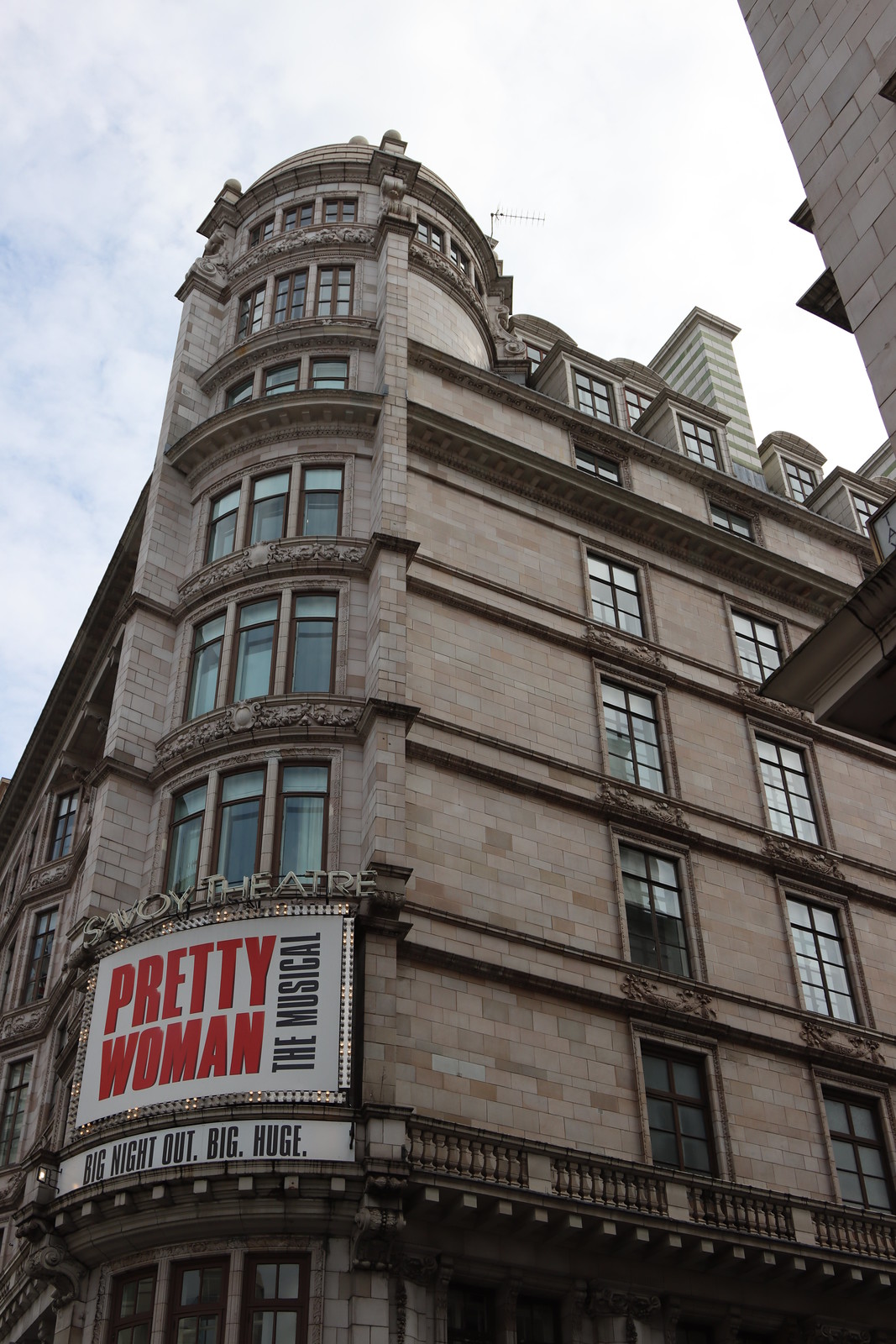The image depicts a grand, historic theater building, eight stories tall, constructed with beige and brown bricks that add to its classical charm. The building, possibly the Savoy Theater, stands prominently at a street corner with its architectural design featuring a turret on the facade. Each floor has a consistent arrangement of three multi-paned windows, with decorative spaces beneath them, creating a symmetrical and aesthetically pleasing pattern on both visible sides of the building.

The central focus is on an eye-catching large white banner above the three main entrance doors. This banner advertises the musical "Pretty Woman" in bold red letters, with "the musical" written vertically in black font alongside it. Below this primary sign is another smaller white banner with the inscription "big night out. big. huge." in smaller black letters, generating excitement for the show.

The image reveals the mix of old-world elegance and vibrant promotional signage, suggesting an intriguing blend of the theater's rich history and contemporary entertainment offerings.